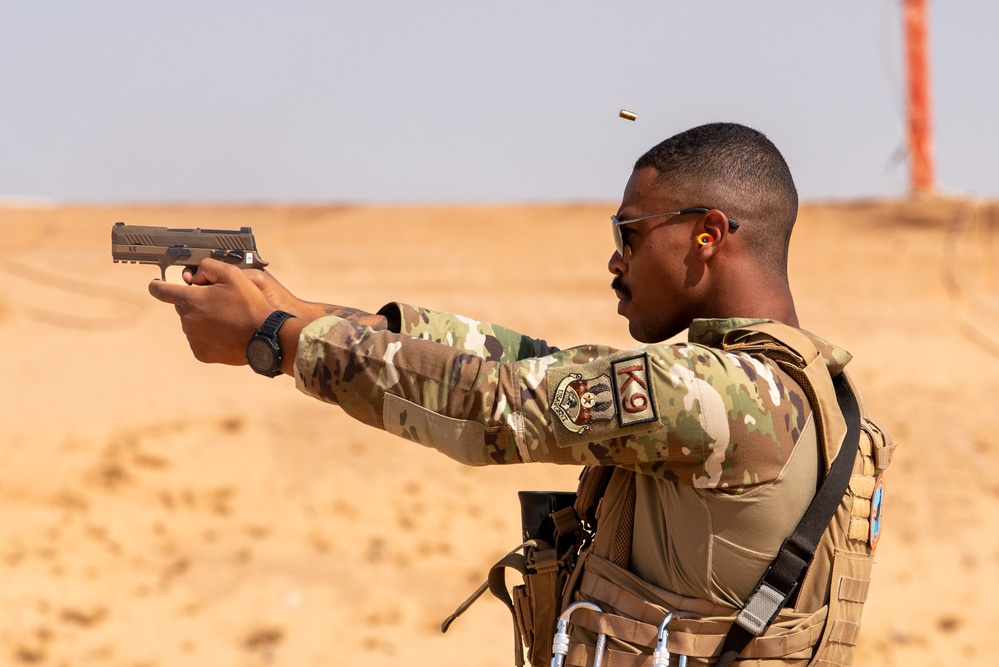The photograph captures an African-American man, estimated to be in his 20s to mid-30s, dressed in a military uniform. His short black hair is cropped close to his head, complemented by a neatly trimmed mustache. He wears a pair of dark sunglasses and red and yellow ear protection. His attire includes a green camouflage shirt beneath a tan tactical vest adorned with carabiners and a black strap crossing his shoulder. Noteworthy patches on his upper left sleeve display the words "K-9" and a distinct insignia.

Positioned with his body turned to the left, he extends both arms to fire a silver gun towards an unseen target. A spent cartridge case is captured mid-air, just above his head. On his left wrist, he sports a black watch. The setting appears to be a desert, evident from the blurred, sandy background and the cloudless sky. An orange pillar, possibly a utility pole, stands in the distance. The image is well-lit, emphasizing the clear, bright conditions of the environment.